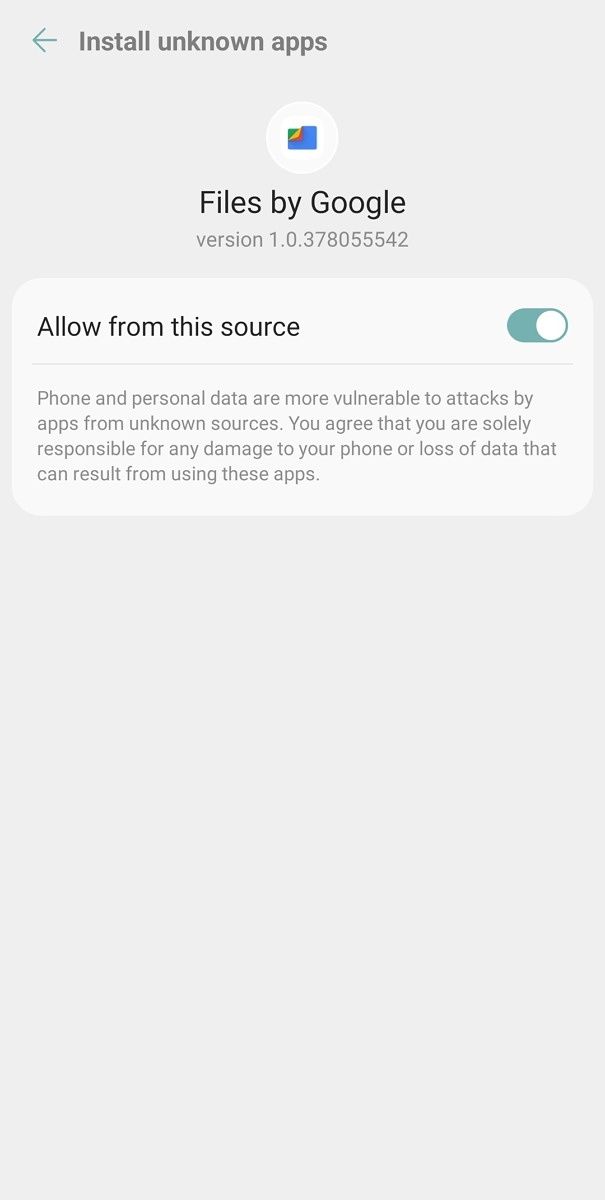The image depicts a settings screen on an Android device dedicated to installing unknown apps. The focus is on the "Files by Google" app, version 1.0.378055542. A prominent toggle switch, labeled "Allow from this source," is set to green, indicating that the option is enabled. Beneath the switch, a cautionary message warns users that their phone and personal data are more vulnerable to attacks from apps obtained from unknown sources. The message emphasizes that users are solely responsible for any potential damage or data loss resulting from using these apps. The screen features a minimalistic design, dominated by a gray color scheme.